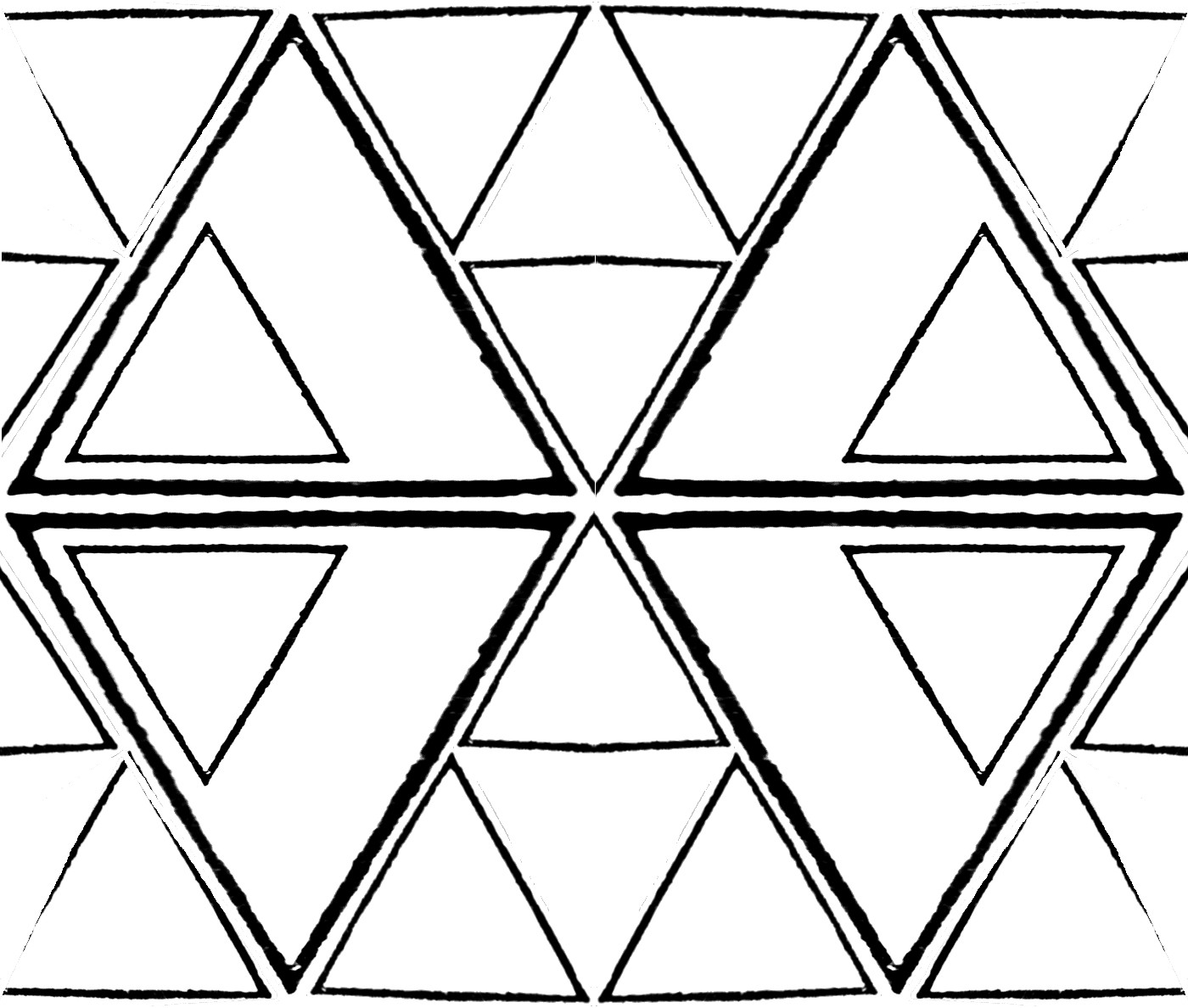This hand-drawn black and white image features intricate geometric patterns formed entirely by triangles. It employs only black ink on a white background, and its artistic complexity is derived from the varying sizes and intersecting arrangements of these triangles. The central focal point of the composition is comprised of four small triangles that converge to shape a larger triangle; these smaller triangles are strategically placed with tiny gaps between their tips. Surrounding this centerpiece is a repeating motif of bold-bordered triangles, each containing smaller, similarly-shaped triangles within them. One prominent pattern involves three upside-down triangles coming together to form a right-side-up triangle in the middle. This configuration recurs across the image, creating a visually engaging tapestry of triangles fitting inside triangles, which collectively give rise to larger, diamond-like formations. The entire image is a testament to the mesmerizing complexity that can be achieved through the simple repetition and rearrangement of a single geometric shape.